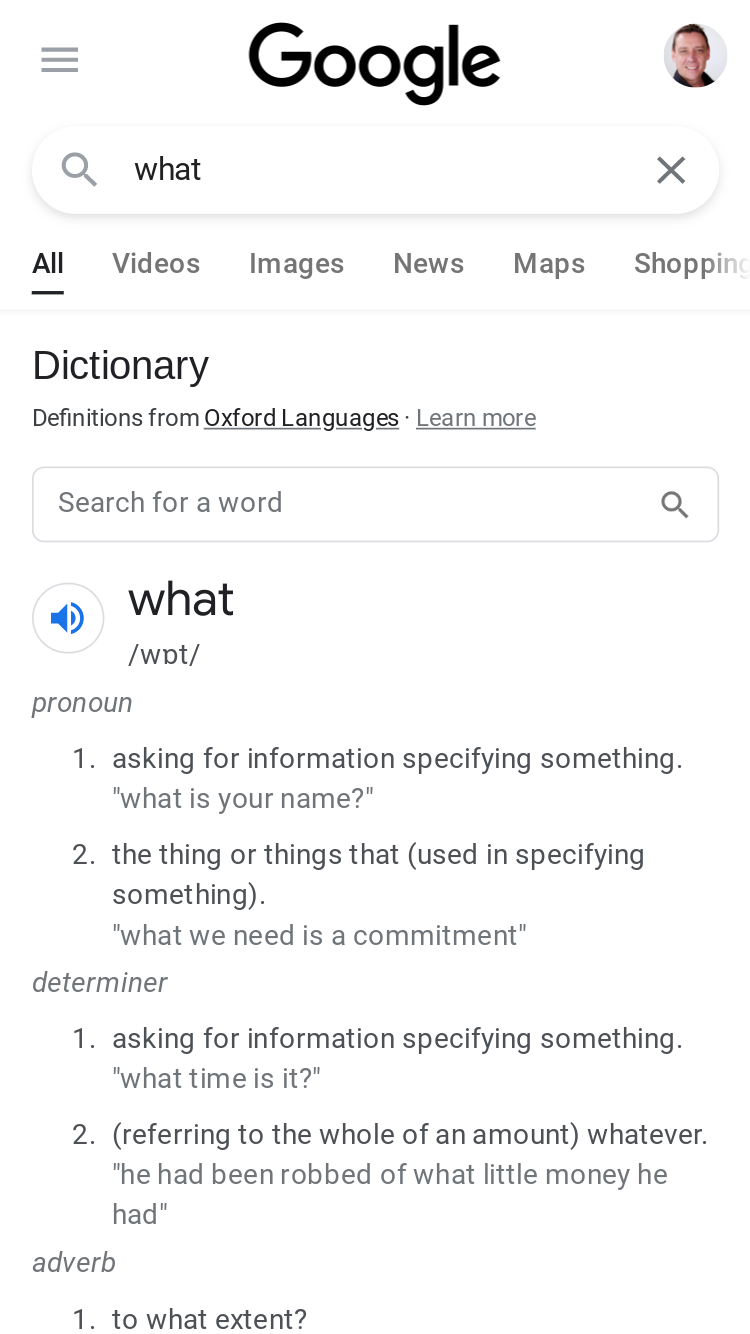The image depicts a Google search page. Prominently displayed in the center is the iconic Google logo in black. To the left of the screen, there's a menu bar represented by three horizontal lines stacked atop one another. On the right side, a circular profile picture featuring the face of a white man is visible. 

Below the Google logo, there's a search bar with placeholder text and a magnifying glass icon on the left and a clear (X) button on the right. Underneath the search bar, navigational options such as "All," "Videos," "Images," "News," "Maps," and "Shopping" are presented. 

Further down, there is a section that reads "Dictionary: Definitions from Oxford Languages - Learn more." Following this, another search bar invites users to "Search for a word" with an embedded magnifying glass icon on the right.

The definition for the word "what" is displayed and described as follows:

**Pronoun**:
1. Asking for information specifying something ("What is your name?")
2. Referring to the thing or things used in specifying something ("What we need is a commitment.")

**Determiner**:
1. Asking for information specifying something ("What time is it?")
2. Referring to the whole of an amount, whatever ("He said that he had been robbed of what little money he had.")

**Adverb**:
1. To what extent ("To what extent?")

The color scheme of the page consists of black, white, gray, blue, and a pinkish-brown skin tone for the profile picture.